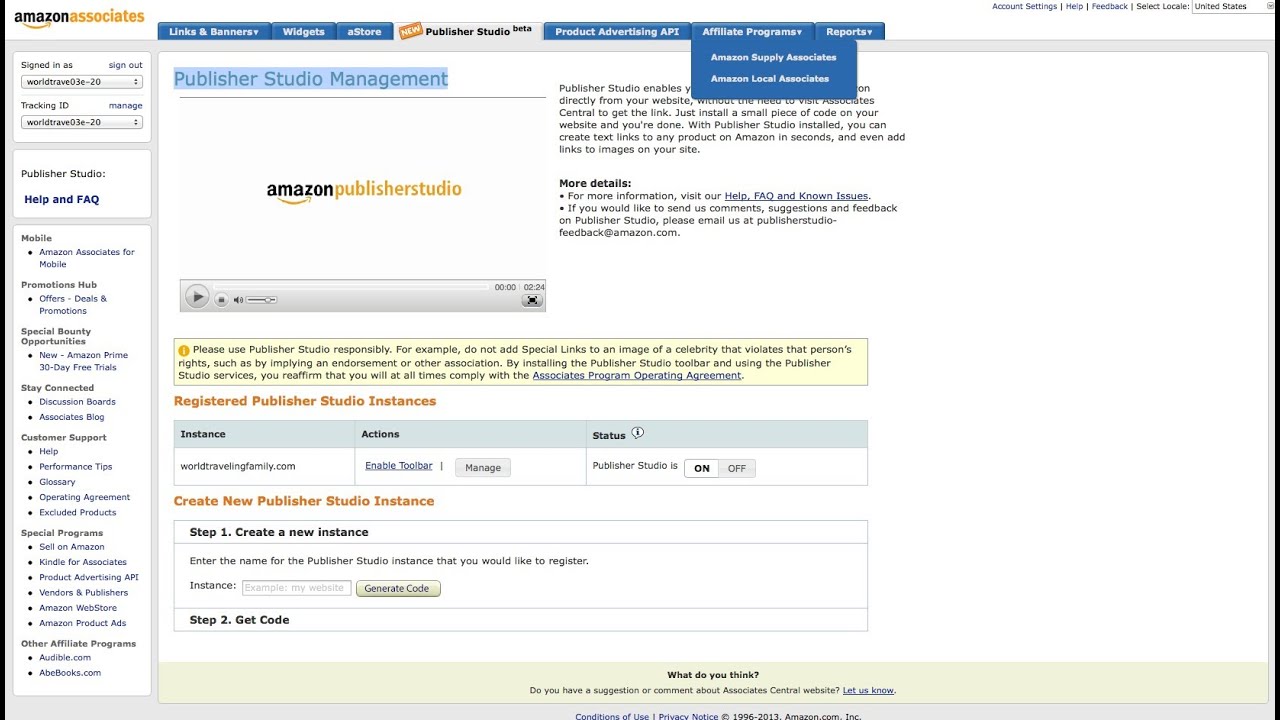The image depicts an Amazon Associates webpage, featuring a variety of links and elements essential for affiliates. Across the top, the page displays categories including Banners, Widgets, E-Store, Publisher Studio, Product Advertising, Art, and the Affiliate Program. 

On the left side of the webpage, users can find the sign-in section, where there is an input field for an ID. Below this, there are several categories such as Publisher Studio, FAQs, Mobile Promotions, Stay Connected, and Customer Help. Each category is neatly organized, providing quick navigation options for users.

The main body of the webpage is dedicated to Publisher Studio Management, highlighted in a light blue color. At the top, "Amazon Publisher Studio" is displayed in Amazon's signature gold and black colors, complete with the iconic arrow underneath the Amazon logo. A clickable link is available to watch an informational video, alongside additional details about the Publisher Studio.

Just below this main section is a yellow bar filled with descriptive text. Further down, there is an area detailing instance actions and status, where users can create new Publisher Studio instances by following the provided guidelines. Towards the bottom of the page, more detailed guidance and instructions can be found, ensuring that users can effectively manage their Amazon affiliate activities.